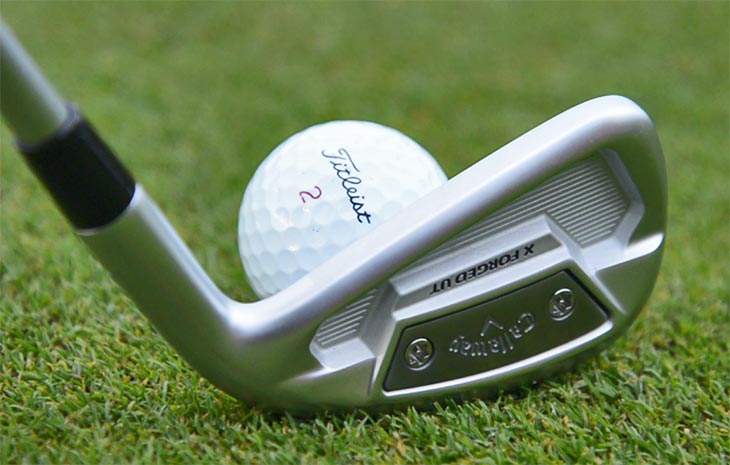This image is a close-up photograph showcasing a Titleist 2 white golf ball positioned on what appears to be green AstroTurf. The concise, neatly trimmed grass foregrounds a silvery-gray X-Forged UT golf club, branded with the name "Callaway," which is engraved and accompanied by one screw on each side of the lettering. The text on the club is shown upside down, making the branding somewhat difficult to read. The golf ball features the distinctive Titleist branding in black lettering accompanied by a red number 2. The club rests at a natural angle beside the ball, suggesting a ready stance but without any indication of movement or the type of shot being set up. The focus diminishes towards the background, making the grass appear blurrier. There are no people or additional context to indicate whether this scene is indoors or outdoors, although the overall impression is one of a meticulously arranged product shot potentially intended for advertising purposes.